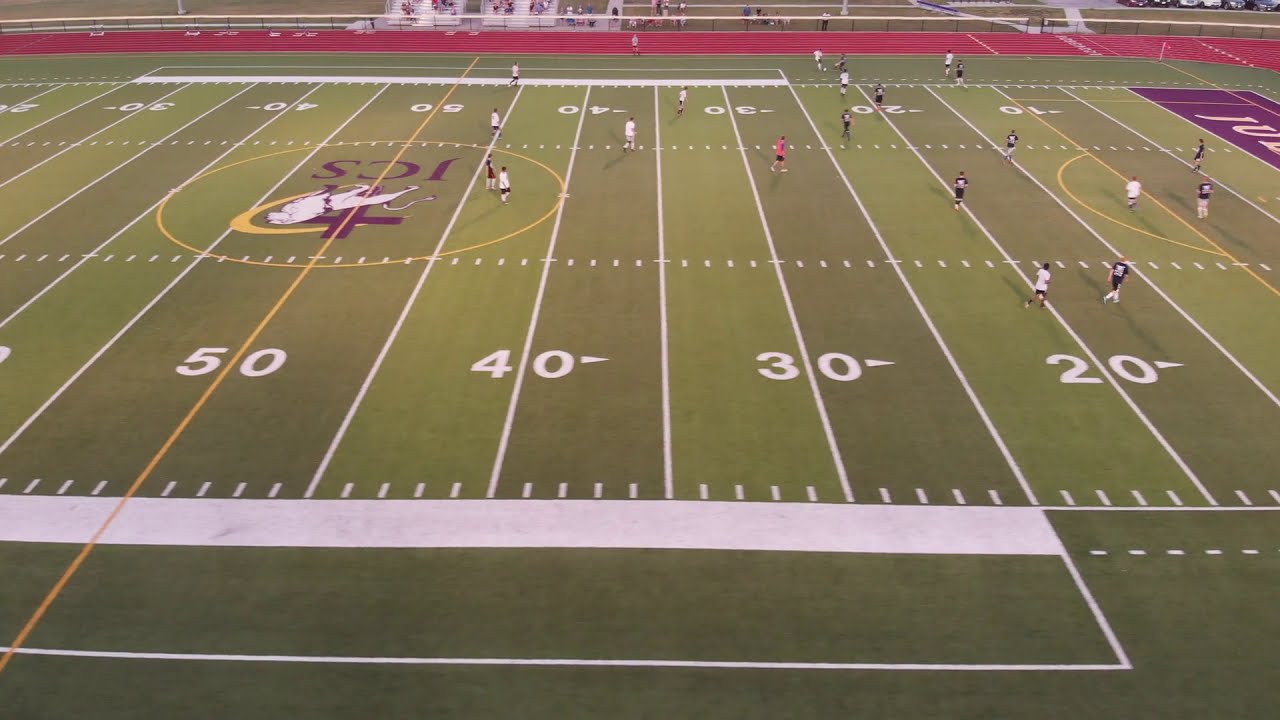This high-resolution image captures a soccer game being played on a football field, likely at a high school given the distinctive emblem at the center. The emblem, upside down from the perspective of the photo, consists of the letters "JCS" in purple alongside a white lion and a cross set in a yellow circle. The photograph spans from the 30-yard line on the left to the distant purple end zone on the right, partially showing the letters "JU." The lush field alternates between lighter and darker shades of green with crisp white yard lines and numbers, including the 50, 40, 30, and 20-yard demarcations. Surrounding the field is a red running track with distant bleachers filled with spectators. On the field, players are distinguished by their white and purple uniforms, accompanied by a referee in a red shirt. The athletes are all dressed in shorts and shirts, confirming that this is a soccer match despite the football field markings.